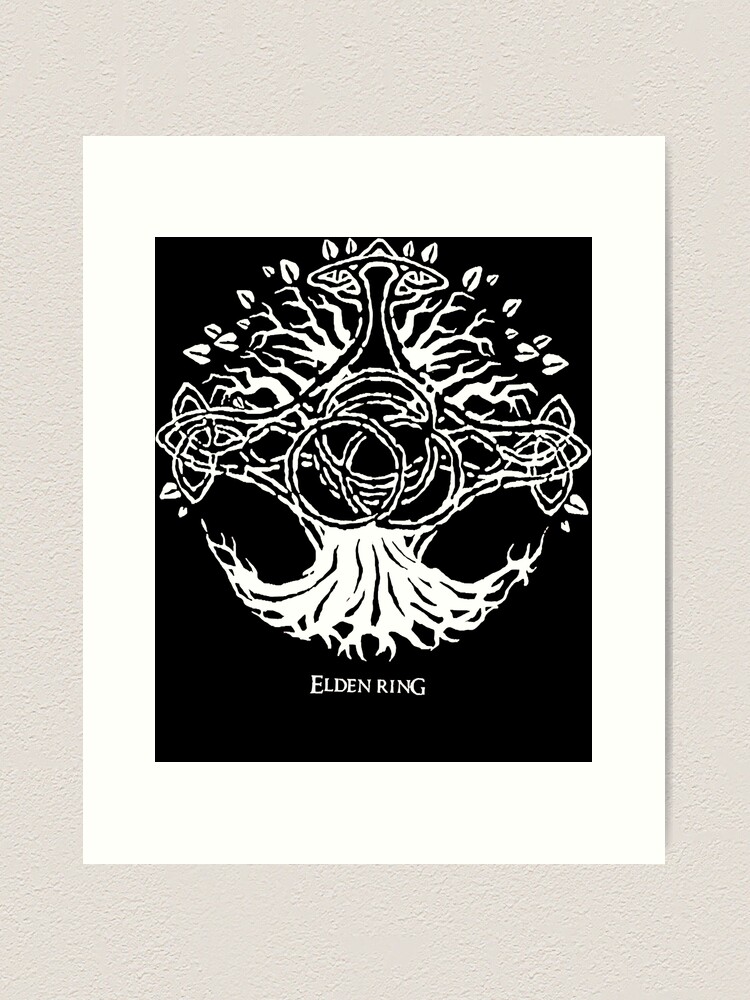The image depicts a stylized black-and-white square painting or print of a tree-like structure. Against a deep black backdrop, the white tree extends its branches outward at the top and fans out its roots at the bottom. The central trunk is adorned with intricate circular patterns, creating an otherworldly and artistic representation rather than a naturalistic one. "Elden Ring" is inscribed in white text beneath the roots. The entire image is mounted on a white, almost cream-colored paper, which contrasts the dark central artwork. Scattered leaves appear to have fallen from the branches, adding further detail to the composition. The aesthetic seems inspired by fantasy motifs reminiscent of J.R.R. Tolkien's Middle-Earth, though it distinctly refers to the Elden Ring universe.